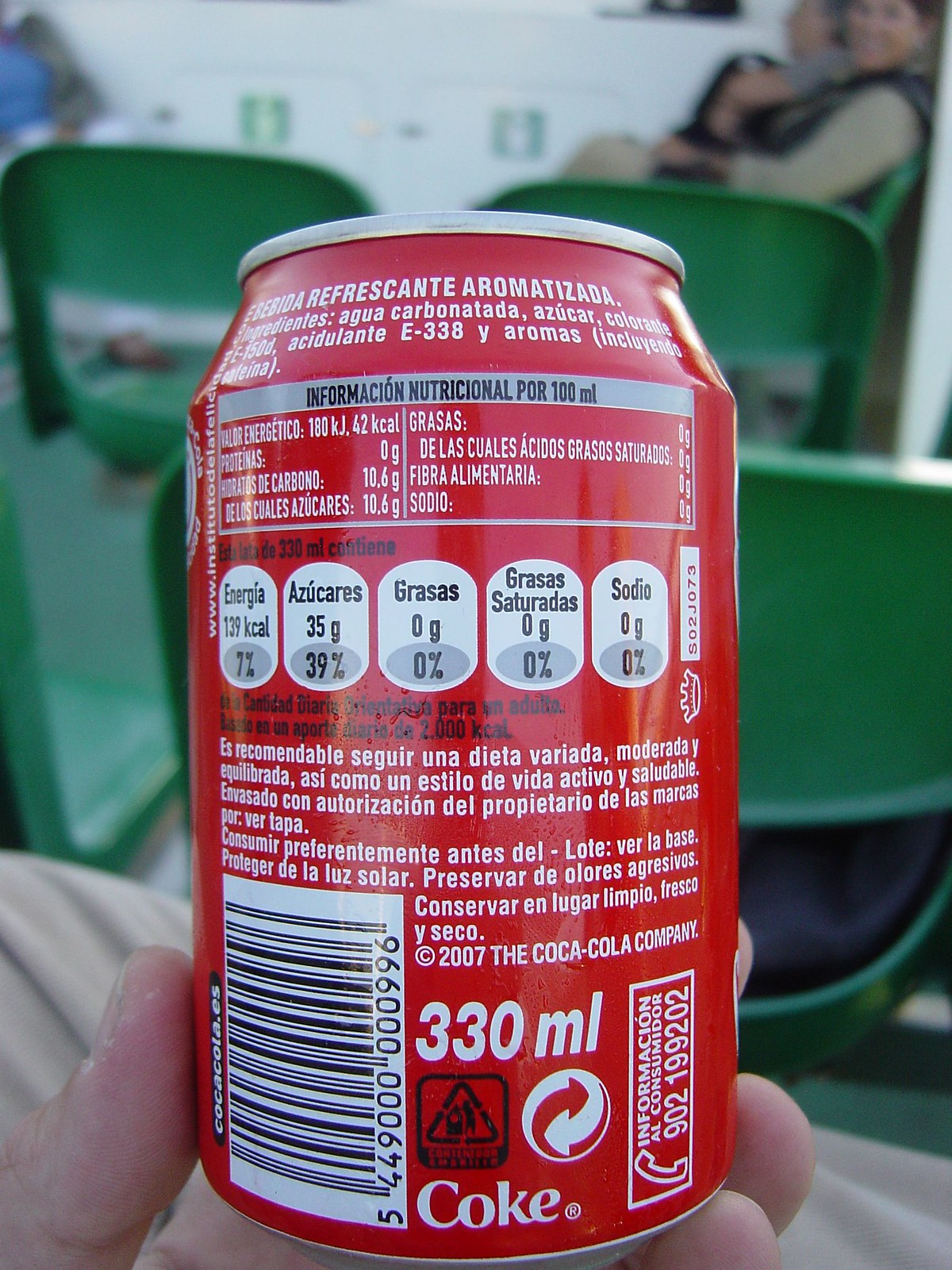In this detailed photograph, a hand delicately holds a standard 12-ounce Coca-Cola can by the fingertips, showcasing the back of the can. The can prominently displays a UPC label and indicates a volume of 330 milliliters. At the bottom, a distinctive Coke logo is visible along with a recognizable recycle symbol. The informational text on the can is entirely in Spanish, adding a unique touch to the image. The background reveals a man tenderly holding a child and includes four green chairs that add an understated yet vibrant contrast to the scene.